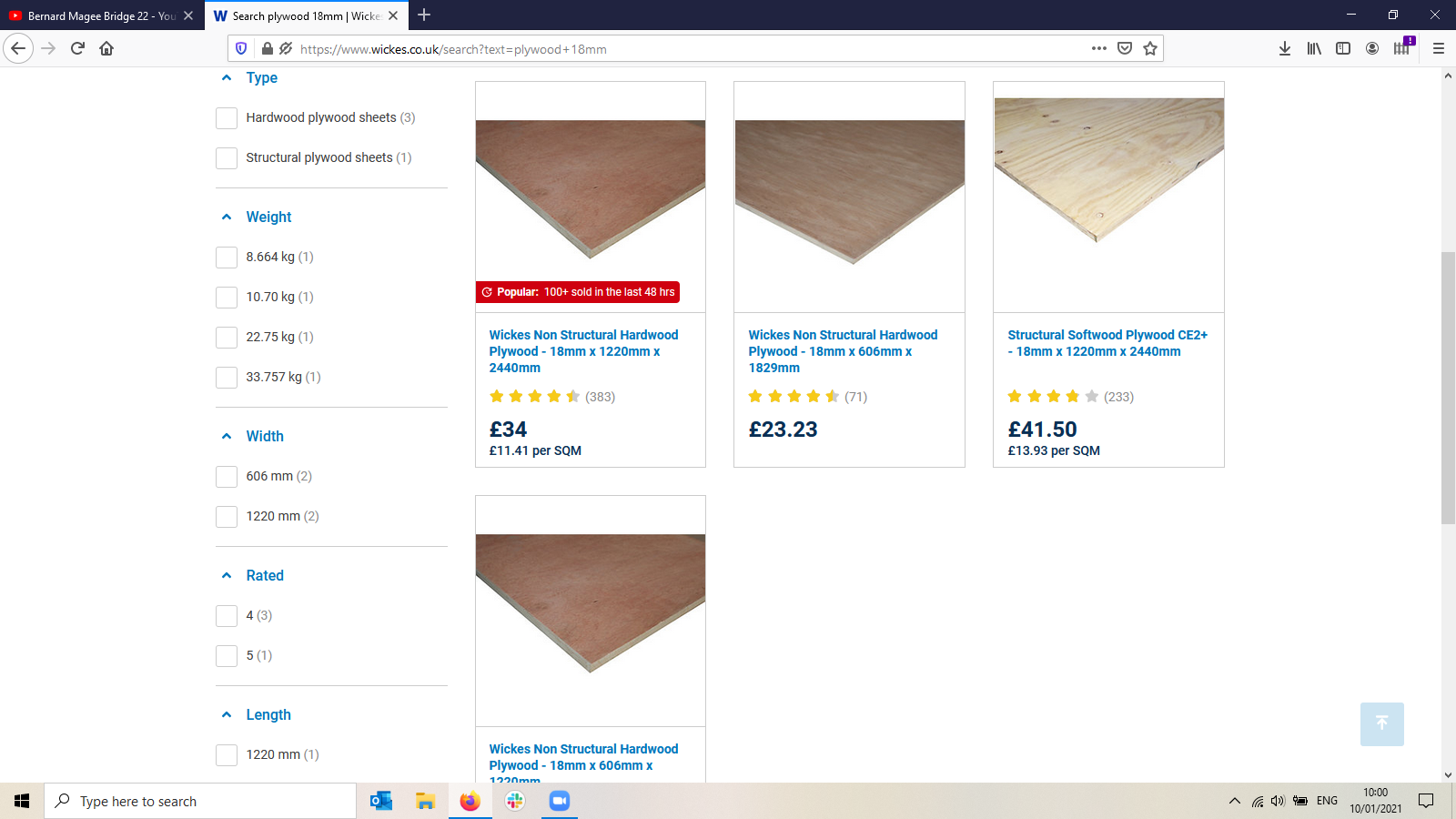**Detailed Image Description:**

The image depicts a zoomed-out view of a web page centered on a hardwood plywood search from an online retailer. The overall layout and intricate details of the page are as follows:

**Top Banner:** 
- The top banner is black with a red logo in the upper left-hand corner. 
- Adjacent to the logo, there is white text reading "Bernard McGee Bridge 22."

**Browser Tabs and Controls:**
- Two tabs are visible. The first tab is labeled "Bernard McGee Bridge 22," and the second tab has a blue "W" icon with text reading "search plywood, 18 millimeter."
- On the top right corner, from left to right, there are the minimize icon, the multiple window icon (indicating an option to enlarge), and the close (X) icon.

**Navigation Bar and Search:**
- Below the tabs, navigation symbols are visible: a back arrow (darkened), a forward arrow (grayed out), a reload icon, and a home icon.
- The address bar includes multiple symbols to the left: a shield icon, a lock, and a strikethrough symbol. The URL displayed is "https://www.wix.co.uk/search?text=plywood+18+millimeters."
- On the right side of the address bar are three horizontal dots, a check mark, a star, and additional icons (a download icon, a stack of books, a square, a silhouette, and a purple box with a track icon, and the menu icon with three horizontal lines).

**Web Page Content:**
- The primary background is white.
- On the left-hand side, filtering options are listed under different categories:
  - **Type:** "Hardwood plywood sheets (3)" and "Structural plywood sheets (1)".
  - **Weight:** Options listed as "8.664 kg (1)", "10.70 kg (1)", "22.75 kg (1)", "33.757 kg (1)".
  - **Width:** "606 mm (2)" and "1220 mm (2)".
  - **Rated:** "4 (3)" and "5 (1)".
  - **Length:** "1220 meters (1)".

**Product Listings:**
- **Product 1:** Wicks Non-Structural Hardwood Plywood, 18 mm by 1220 mm by 2440 mm, reddish brown, rated 4.5 stars (383 reviews), priced at 34 pounds (11.41 pounds per square meter).
- **Product 2:** Wicks Non-Structural Hardwood Plywood, 18 mm by 606 mm by 1829 mm, tan, rated 4.5 stars (71 reviews), priced at 23.23 pounds.
- **Product 3:** Structured Softwood Plywood, CE2+, 18 mm by 1220 mm by 2440 mm, light oak tan, rated 4 stars (233 reviews), priced at 41.50 pounds (13.93 pounds per square meter).
- **Product 4:** (Partially cut off) Wicks Non-Structural Hardwood Plywood, 18 mm by 606 mm by 1220 mm.

**Taskbar Details:**
- Visible on the taskbar are the Windows icon, a search bar, Outlook, a file icon, Mozilla Firefox browser icon, an unidentified icon that might resemble an old Chrome logo, and a video camera or Zoom icon.
- On the far right of the taskbar, you can see the Wi-Fi signal, a speaker icon, a charging battery indicator, the language setting ("ENG"), the time (10:00 AM), and the date (October 1, 2021).